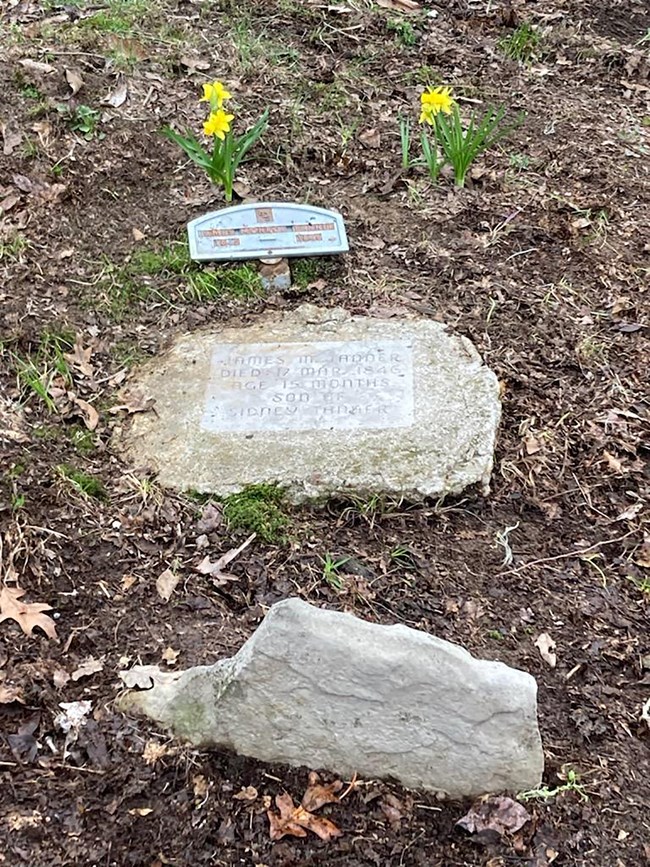A weathered, old gravestone lies amidst a sparse, untended area filled with dry leaves, dirt, and sporadic patches of grass. The grave marker is a stone slab with an etched or attached stone plaque that is hard to decipher due to age and dirt. The plaque faintly reads James M. Tadder, who died on March 17th, 1846, at the age of 15 months, son of Sydney Tadder. Behind this marker is another, smaller, bluish plaque with illegible writing. In front of the gravestone, there is a sharp, protruding rock, roughly the size of the gravestone itself. Flanking the gravestone are two daffodil plants with yellow flowers, their vibrant colors standing out against the muted, earthy surroundings. The setting suggests a grave not in a typical cemetery but rather in a more secluded, overgrown area.